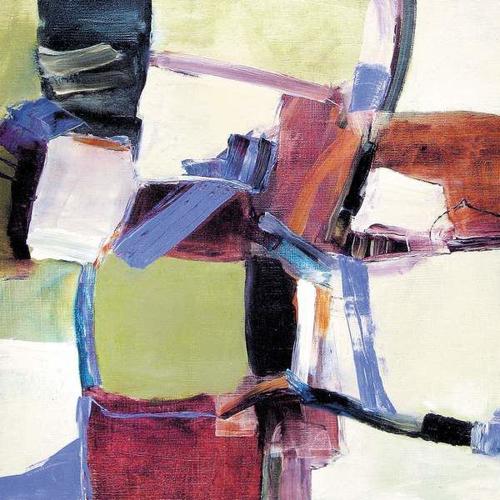This image is a rectangular piece of abstract art, slightly taller than it is wide, featuring an eclectic mix of colors and materials that come together in a seemingly chaotic, yet intriguing composition. The color palette is subdued, consisting of pea greens, periwinkle blue, muted orange, muted pink, cream, a darker red-purple, black, and white. The artwork incorporates geometric shapes that are noticeable yet imperfect, with square-ish and rectangular forms that appear incomplete. The colors and shapes might evoke natural elements like grass, water, or crops, but this interpretation is open to the viewer's perspective.

The image also seems to blend different media, resembling torn fabric strips of various sizes, some of which are maroon and white. This fabric appears to be intertwined with either tape or paint, making it hard to distinguish the exact materials used. The background is predominantly white, which helps to highlight the colorful, random brush strokes and the textured layers created by the fabric and paint or tape. It gives the impression of a child’s whimsical creation but holds an underlying complexity that invites deeper contemplation, blending the abstract with a modernist cubist influence.